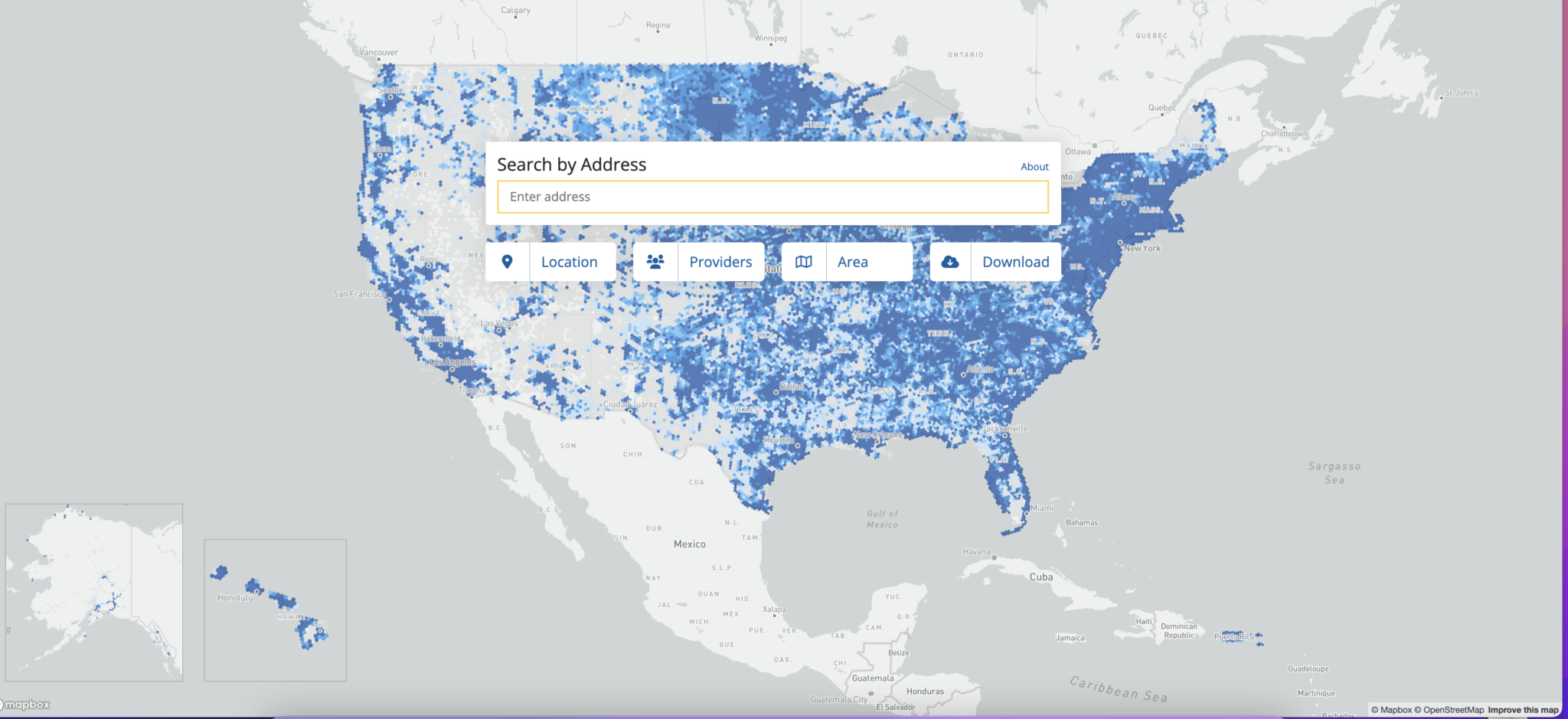This screenshot appears to depict a detailed map illustrating cell phone coverage across various regions, primarily focused on the United States. In the bottom left corner, there's a map of Alaska, predominantly white with some blue areas, indicating coverage zones. Next to it, Hawaii is shown with most islands in blue, except the largest island which is white. Surrounding these maps is the vast blue expanse of the Pacific Ocean on the left and the Atlantic Ocean on the right.

Centrally located on the map, Canada is shaded in gray, and the United States is displayed with a spectrum of blue hues. The darker blues signify stronger coverage areas, while lighter blues represent weaker coverage, and white areas denote lack of coverage. Directly south of the United States are Mexico and Cuba, which are depicted within the Caribbean waters.

At the top center of the screenshot, there's a white search box with "Search by address" written in black text. Below the yellow bar within the search box, it says "Enter address" in gray. Further down, four buttons are visible against a white background labeled "Location," "Providers," "Area," and "Download," each highlighted in blue.

Considering the elements presented, this screenshot likely represents a cell phone coverage map, where the various shades of blue indicate coverage strength, and white areas represent no coverage. This map is possibly used to check cell phone signal availability across different geographical locations.